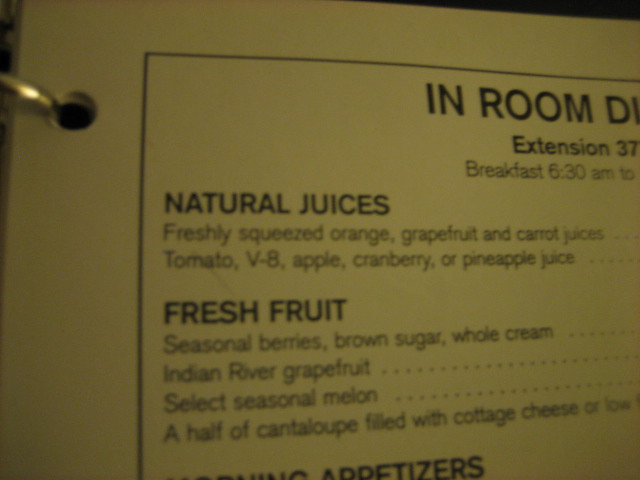Close-up of an in-room dining menu page from a hotel or bed and breakfast, held in a ring binder with the top hole and silver ring clearly visible. This menu is likely part of the comprehensive welcome book that details all about the hotel amenities and surrounding area. Though prices aren't visible, they likely reflect the high-end offerings typical of such establishments. The menu heading reads "In-Room Dining" with a visible extension number for ordering. Breakfast service is available from 6:30 AM onwards, though the exact end time is not shown. 

In capitalized, bold black letters, the menu highlights "Natural Juices," followed by a list of freshly squeezed options including orange juice, grapefruit juice, carrot juice, V8 tomato juice, apple juice, cranberry juice, and pineapple juice—ensuring a delightful variety for all tastes.

Under "Fresh Fruit," the offerings include seasonal berries with brown sugar and whole cream, Indian River grapefruit, select seasonal melon, and an intriguing dish of half a cantaloupe filled with cottage cheese. The detailed and diverse selection promises something for every palate.